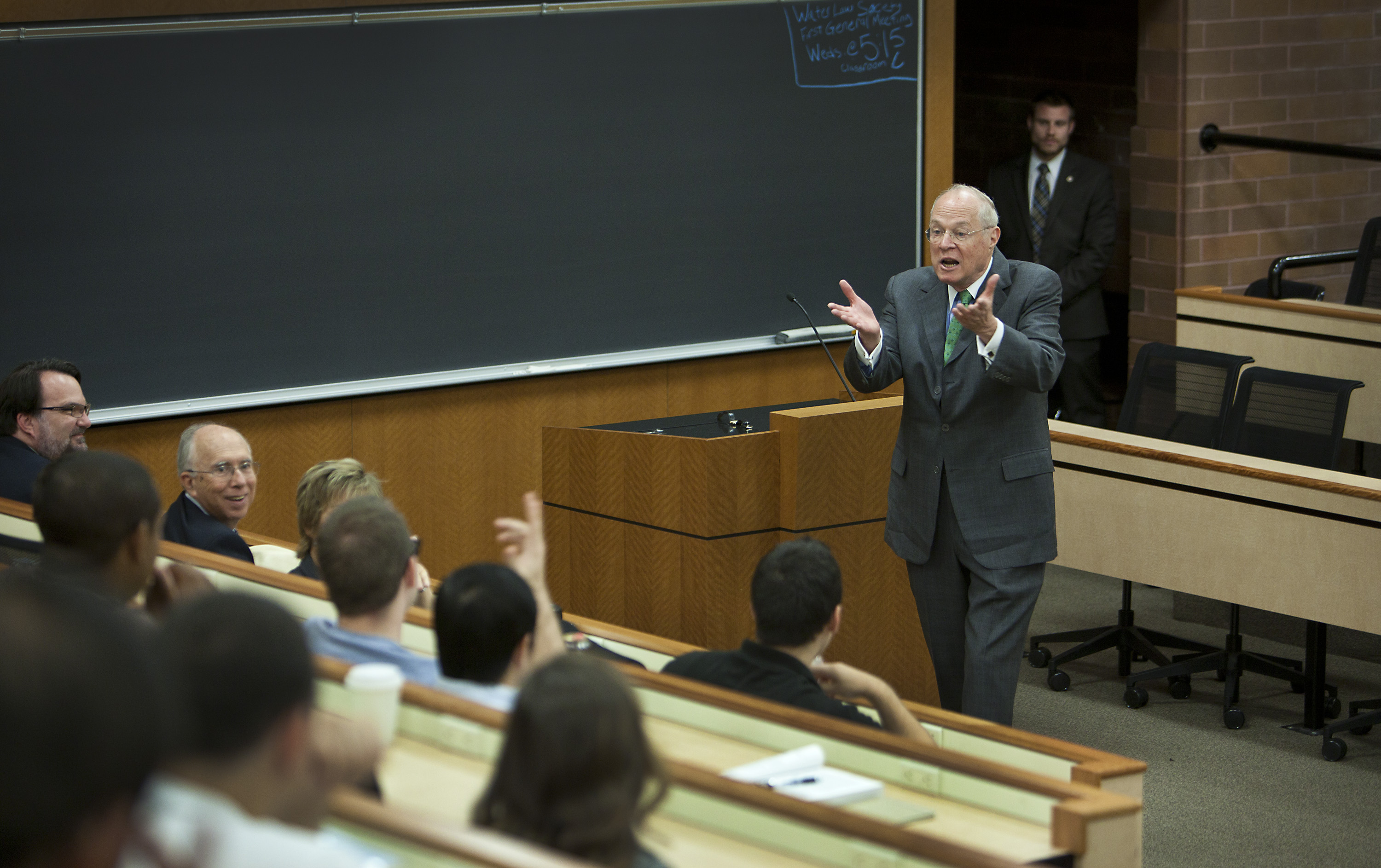In the photograph, we see the interior of a brick-walled classroom with tiered seating, ensuring everyone has a clear view. The long thin tables on each side of the room rise from the floor upwards. A prominent long chalkboard spans one side of the room. At the forefront, an older gentleman with white hair, wearing glasses and a medium gray suit, stands behind a podium equipped with a microphone. He is actively engaged in speaking to the 10 male students, his arms raised halfway with palms up, indicating an emphasis in his speech. Among the students, one man has his hand raised, appearing ready to ask a question. In addition, a man in a dark suit and white shirt stands attentively in the doorway, while another individual in a brown suit with a beard and mustache stands behind the speaker in the background. The mood suggests a dynamic and interactive lecture, possibly during a class or conference.